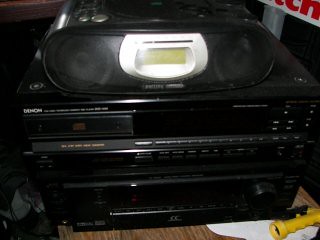The image features a visually intricate setup of audio equipment placed atop a light brown wooden table. At the center is a multi-component stereo system, which appears to consist of three distinct units stacked on top of each other. Each unit is black with various buttons and switches, some large and others small, interspersed with unreadable white lettering. 

At the top of the stack sits a compact, old-fashioned boombox. The boombox features a prominent silver accent in the middle, with a digital screen centrally positioned within this silver section. Flanking the silver center are small speaker grills on either side. Below the boombox, one of the stereo units contains what seems like a cassette deck, marked with a silver area reminiscent of classic tape players. The bottom-most unit is suggested to potentially have a CD player, identifiable mostly by its muted outline.

The table also holds a yellow hose end wand with a black handle, resting on a white cloth. In the backdrop, a metal post with a white sign displaying red, indistinguishable lettering is faintly visible, alongside another brown table. The overall scene depicts a blend of vintage and utilitarian elements in a home setting.